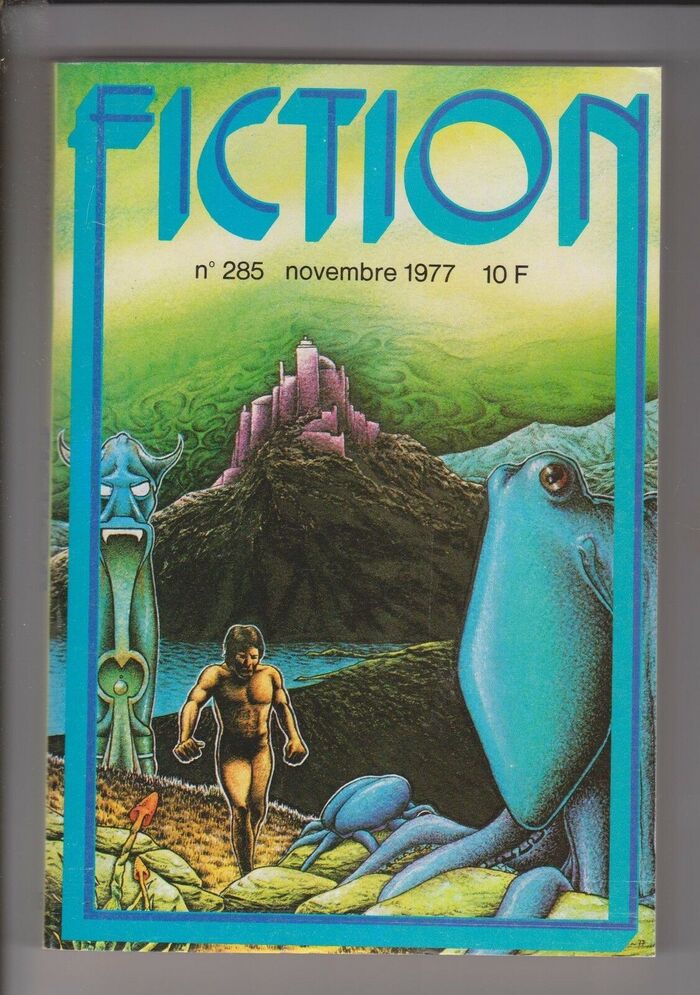This image is a detailed, vintage-style color illustration that appears on the cover of a magazine or comic book from November 1977. The magazine title "FICTION" is prominently displayed at the top in bold blue letters with an aqua drop shadow, extending from the 'F' and 'N' to create a frame around the artwork. The background of the magazine is predominantly green in varying shades, set against a gray backdrop. 

Central to the illustration is a purple, castle-like structure perched on a large brown hill, which descends to a thin strip of blue water and another smaller brown hill below. Text in black letters below "FICTION" reads "N° 285 Novembre 1977 10 F". To the left of the castle, there is a devilish creature with horns and a long tongue reaching downward, painted in shades of green. 

In the foreground, a yellow-skinned caveman figure, appearing naked, walks toward the right side of the image. To the far right, a blue octopus with a single eye peers out at the viewer, its tentacles spread across the corner. Additional details include a few flowers and rocks at the bottom left, enhancing the painted, illustrative style of this aged magazine cover.